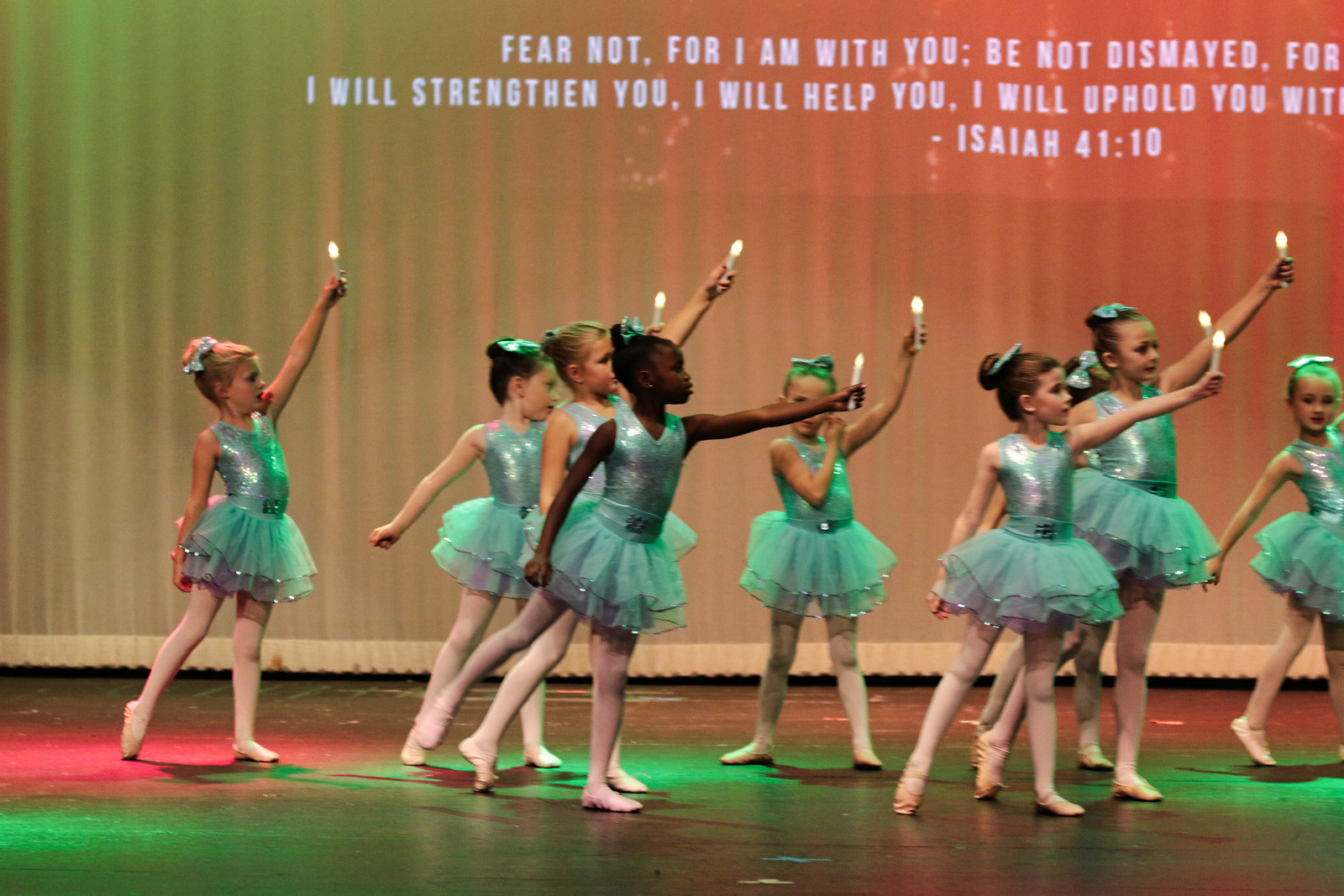In the photograph, a group of young girls, dressed as ballerinas in light green tutus, are positioned in the center of the image. They are performing on a stage with a hard floor, illuminated by green stage lights and a hint of red light on the left. Each girl holds an electronic candle in her outstretched left arm, mostly facing right. Their hairs are styled in buns, adorned with ties. The background features a striped green and orange curtain, with some tan coloring, and text projected onto it. The text reads: "Fear not, for I am with you; be not dismayed, for I will strengthen you, I will help you, I will uphold you,” a quote from Isaiah 41:10. One girl in the center faces the camera with her arm partially obscured by another performer. The setting suggests they are in the midst of a dance recital or performance in an indoor venue.